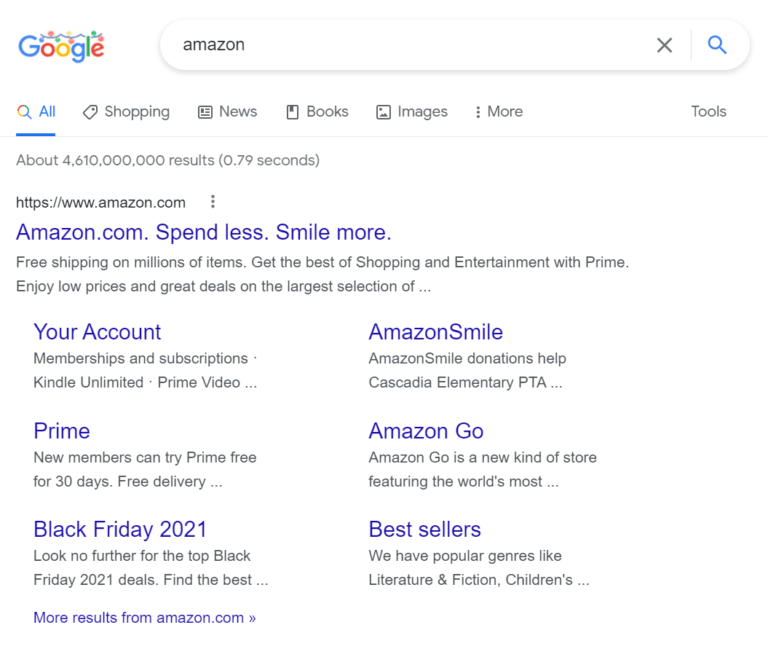A screenshot of the Google search engine webpage is displayed, capturing a search query for "Amazon." Dominating the upper portion is the iconic Google logo on the left, accompanied by the central search bar where "Amazon" is typed. Below the search bar, a horizontal menu presents various search categories such as All, Shopping, News, Books, Images, and More. 

The first prominent search result is Amazon's official website, identified by the URL www.amazon.com in small text beneath a hyperlink to the main site. A brief description follows, stating "Free shipping on millions of items. Get the best of shopping and entertainment with Prime. Enjoy low prices and great deals on the largest selection of." 

Additionally, the search result includes direct links to Amazon's subcategories like "Your Account," "Prime," "Black Friday 2021 Sales," "Amazon Smile," "Amazon Go," and "Best Sellers," each accompanied by a concise informative description. The entire page is set against a clean, white backdrop, ensuring readability and focus on the search content.